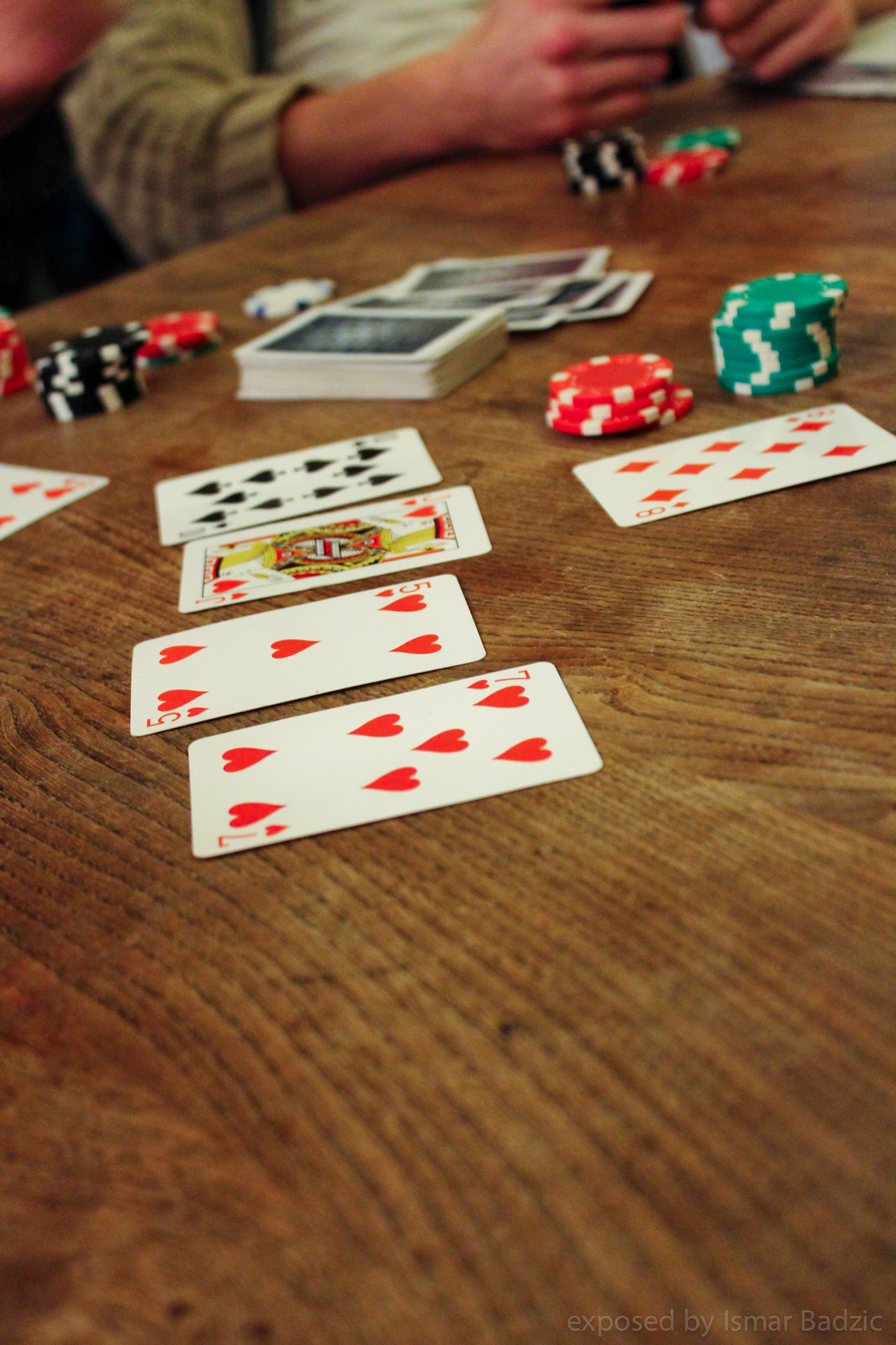In this photograph, a rich tableau of a poker game is spread out on a brown table. Prominently displayed are playing cards: a seven of hearts in the forefront, followed by a five of hearts, a king, and a card from the clubs suit, whose number is obscured. To the upper right, a six of diamonds is visible, adjacent to stacks of poker chips in red and white, and green and white, with the green and white chips forming a taller stack. Behind these chips lies a substantial pile of roughly 30 more cards. Additional poker chips in black and white, red and white, and a distinctive white chip with blue squares are distributed across the table.

In the far corner, a person’s forearms and hands are visible, resting on the table. They are dressed in a gray sweater and have several poker chips positioned directly in front of them, including black and white, red and white, and green and white variations. The scene evokes the tense, anticipatory atmosphere of a high-stakes poker game.